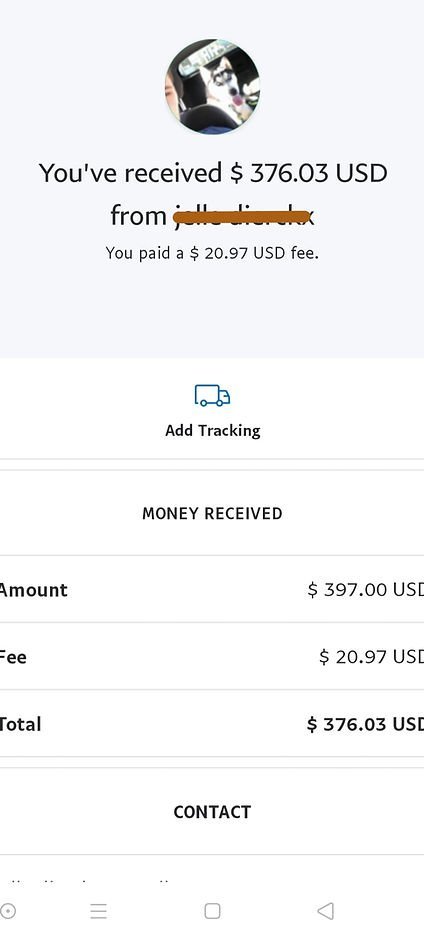The image is a screenshot of a smartphone displaying a money transfer app interface. At the top, there is a small profile picture partially showing a person's face, but the main focus is on a dog situated behind them. The screen indicates that $376.03 USD has been received from an individual whose name is crossed out. A notification highlights that a $20.97 USD fee was paid for the transaction. Below this, there's an option to add tracking, represented by an icon of a truck.

The details of the transaction are listed clearly: the amount received is $397 USD, with a deducted fee of $20.97 USD, resulting in a total of $376.03 USD. An option to contact the sender is available underneath the transaction details. At the very bottom, a menu bar features several icons: a circle with a dot inside it, three horizontal lines stacked together, a square, and a triangle or arrow pointing to the left. The background is entirely white, and all text is in black, ensuring clear visibility.